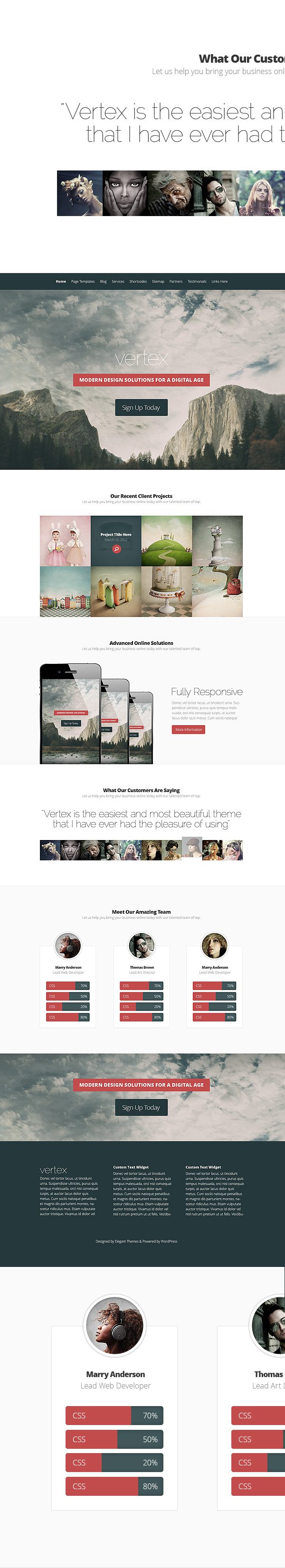**Caption:**

This image features a promotional poster for "Vertex: Modern Design Solutions for a Digital Age." The poster invites viewers to sign up and showcases several recent client projects. Despite the image being somewhat blurry, certain elements are discernible. Prominently displayed are two China dolls dressed in rabbit fur capes and hats with bunny ears, exuding a cute aesthetic. In the background, there's a green box with the placeholder text "Project Title Here," and a red circle containing a key symbol. One section of the poster shows a verdant mound with a pathway leading up to the top, surrounded by trees and a fence, suggesting a scenic landscape.

Further details include an intriguing setup where a bag of gold coins appears to support a light system by the ocean, illuminating a gray structure with light on its top, near a sandy beach. The poster also contains a text endorsing Vertex’s theme as being beautiful and easy to use, attributed to customer testimonials.

Additionally, various images enrich the poster: a sideways clown, a person cradling their cheeks with their hands, an eerie elderly woman, a person apparently using an iPad, a warrior girl, an AI girl with black hair, a woman resembling Lady Bird Johnson wearing virtual reality goggles, and a girl with a racing cap and long hair. Testimonials from individuals such as Mary Anderson and Thomas Brown highlight the team behind Vertex, reiterating the advanced online solutions and fully responsive design that the company offers.